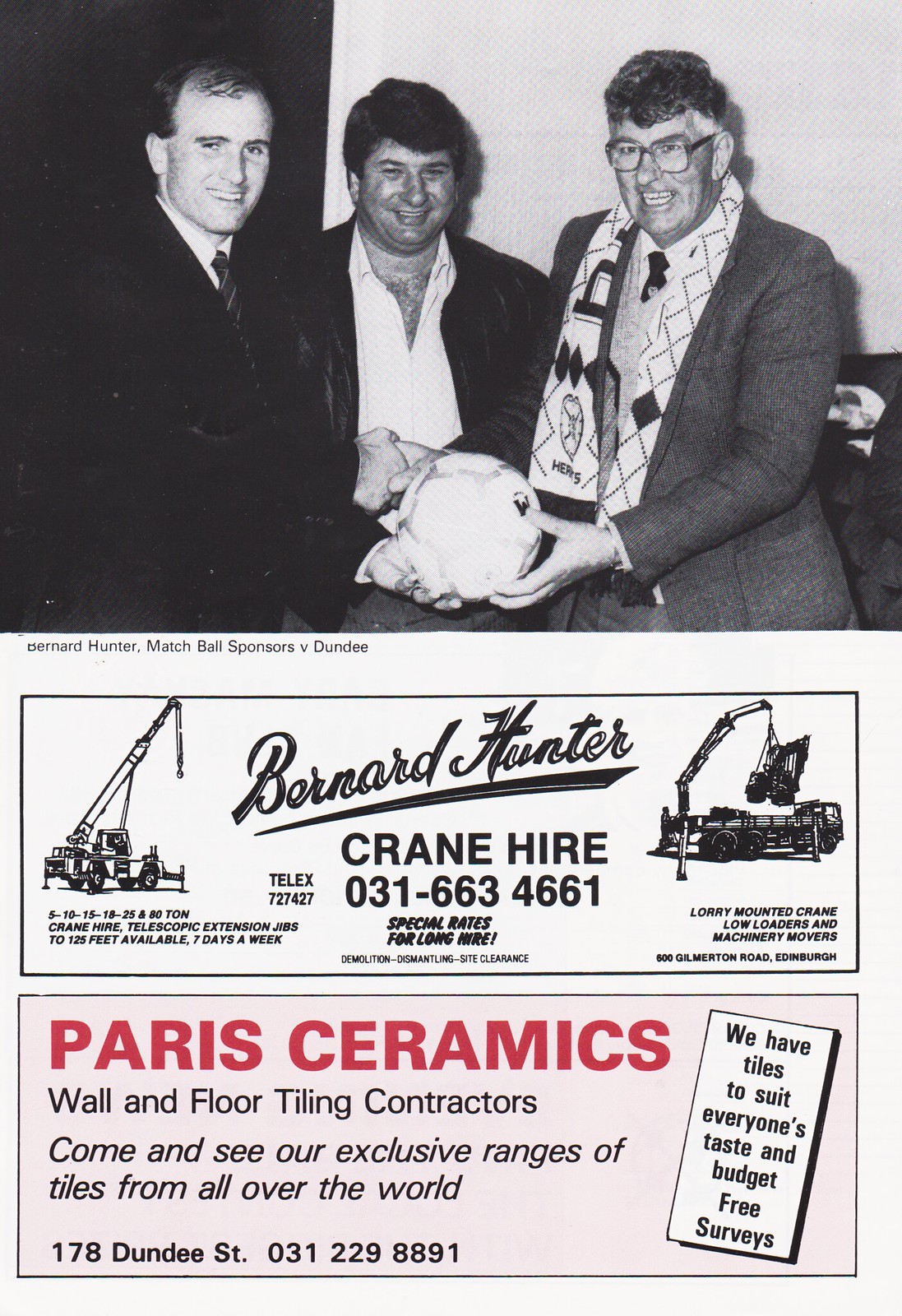The image resembles an advertisement page from an older phone book or magazine, divided into three distinct sections. The top half features a black-and-white photograph of three men, identified as the Bernard Hunter match ball sponsors for a game against Dundee. The men, dressed in varying styles of jackets and suits—one with a more casual open shirt, another wearing glasses and a scarf—are shaking hands and collectively holding what appears to be a soccer ball. Directly below their photo is an advertisement for Bernard Hunter, Crane Hire, listing a phone number (031-663-4661) and featuring small black stencil drawings of cranes to emphasize their services. Further down, occupying a light pinkish rectangle with bold red lettering, is another advertisement for Paris Ceramics, Wall and Floor Tiling Contractors, providing their address at 1778 Dundee Street and phone number (031-229-8891).